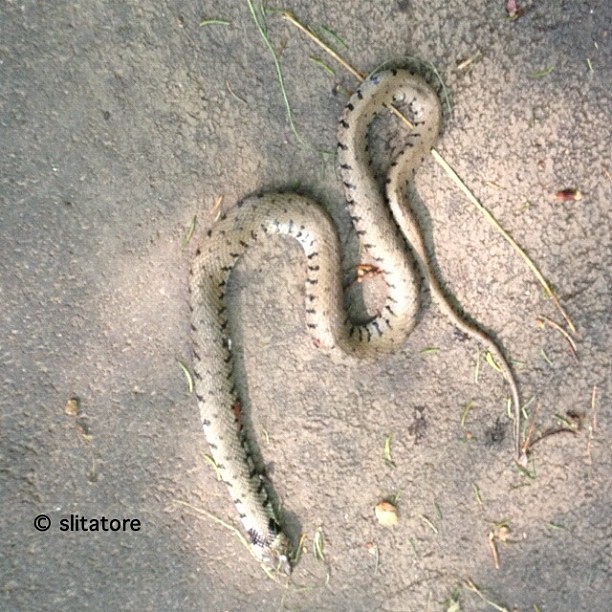The image depicts a light gray snake, approximately six feet long, positioned on a grainy, barren ground that resembles either a beach or a concrete surface. The snake, appearing to be either deceased or feigning death, is lying on its back, displaying a white belly with dark speckles and black stripes. Its body forms a coiled S-shape, while a few pieces of grass and vegetation are scattered around it. The background is predominantly barren with little to no foliage. In the lower left-hand corner of the image, there is a black text reading "Slithator" with a copyright symbol next to it. The scene is minimalistic with only a few stems of plants and grasses visible, emphasizing the lifeless or defensive posture of the snake on the desolate ground.